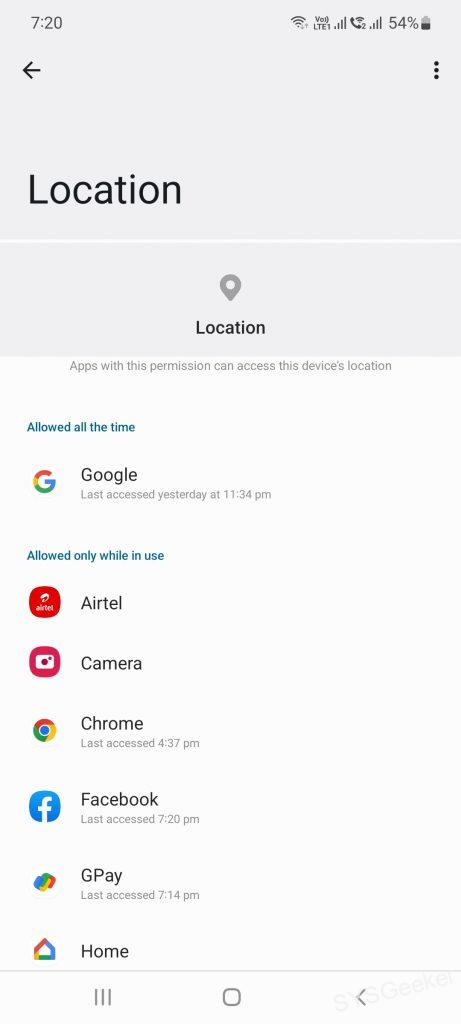This image captures a screenshot of an Android smartphone's location settings screen. The status bar at the top indicates that the time is 7:20, and the battery level is at 54%. On the upper left is a back button, while the upper right features a three-dot menu button. 

The screen's header is gray, featuring a location pin icon with the word "Location" next to it. Below, it reiterates "Location" and explains that "Apps with this permission can access this device's location." 

The list below is segmented into apps that are "Allowed all the time" and those that are "Allowed only while in use." For the apps that are "Allowed all the time," Google is listed with its rainbow 'G' icon, noting it was last accessed yesterday at 11:34 PM.

Under "Allowed only while in use," several apps are listed:
- Airtel, indicated by a red icon.
- Camera, marked with a pink icon featuring a camera symbol.
- Chrome, represented by its colorful red, yellow, and green circle with a blue center, last accessed at 4:37 PM.
- Facebook, illustrated with its blue 'F' logo, which was last accessed at 7:20 PM.
- GPay, shown as a rainbow-colored cloud, last accessed at 7:14 PM.
- Google Home, denoted by a home icon.

The subsequent apps in this list are not visible in the screenshot.

At the bottom of the screen, there are three navigation buttons: a menu button, a back button, and another function button. The overall background of the image is white and gray, contributing to a clean and minimalistic design of the setting screen.